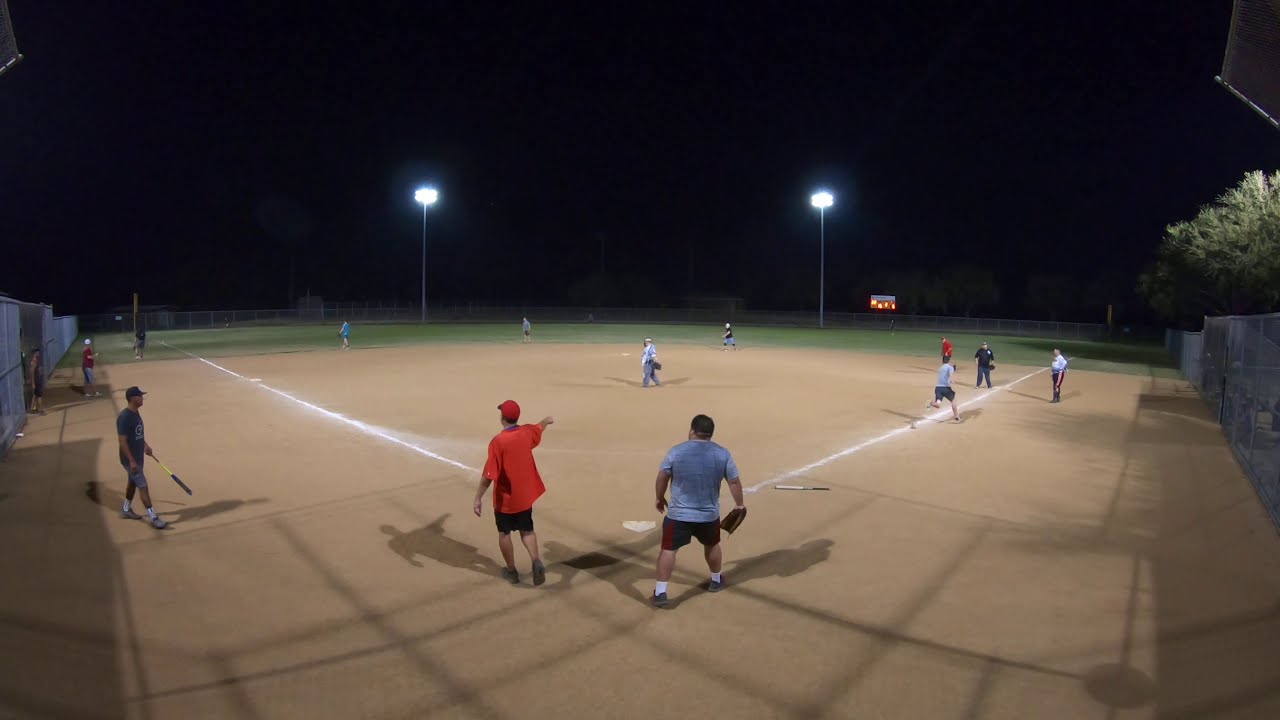This captivating nighttime photograph captures an adult softball game in full swing under a black sky. The scene is illuminated by two tall light stands positioned in right and left center fields, casting a bright glow over the green outfield grass and the light tan clay of the infield. A fence encircles the entire field, with a lit scoreboard visible in left center, displaying the game’s tally.

At home plate, a blue-shirted catcher with a mitt is stationed, ready for action, and another notable figure in a red shirt and cap is pointing towards something, possibly officiating the game. Nearby, a player in a gray shirt and shorts, streaked with sweat, is seen at bat, while another batter in a gray shirt is rounding first base, indicating a recent hit. The yellow and black bat they used lies near the first base line.

Players are strategically positioned on first, second, and third bases, contributing to the dynamic energy of the ongoing game. The outfield has multiple players ready to field the ball, completing the bustling scene surrounded by trees along the park's right side. The cohesive details from various perspectives narrate the unfolding drama of an exciting baseball game under the night sky.